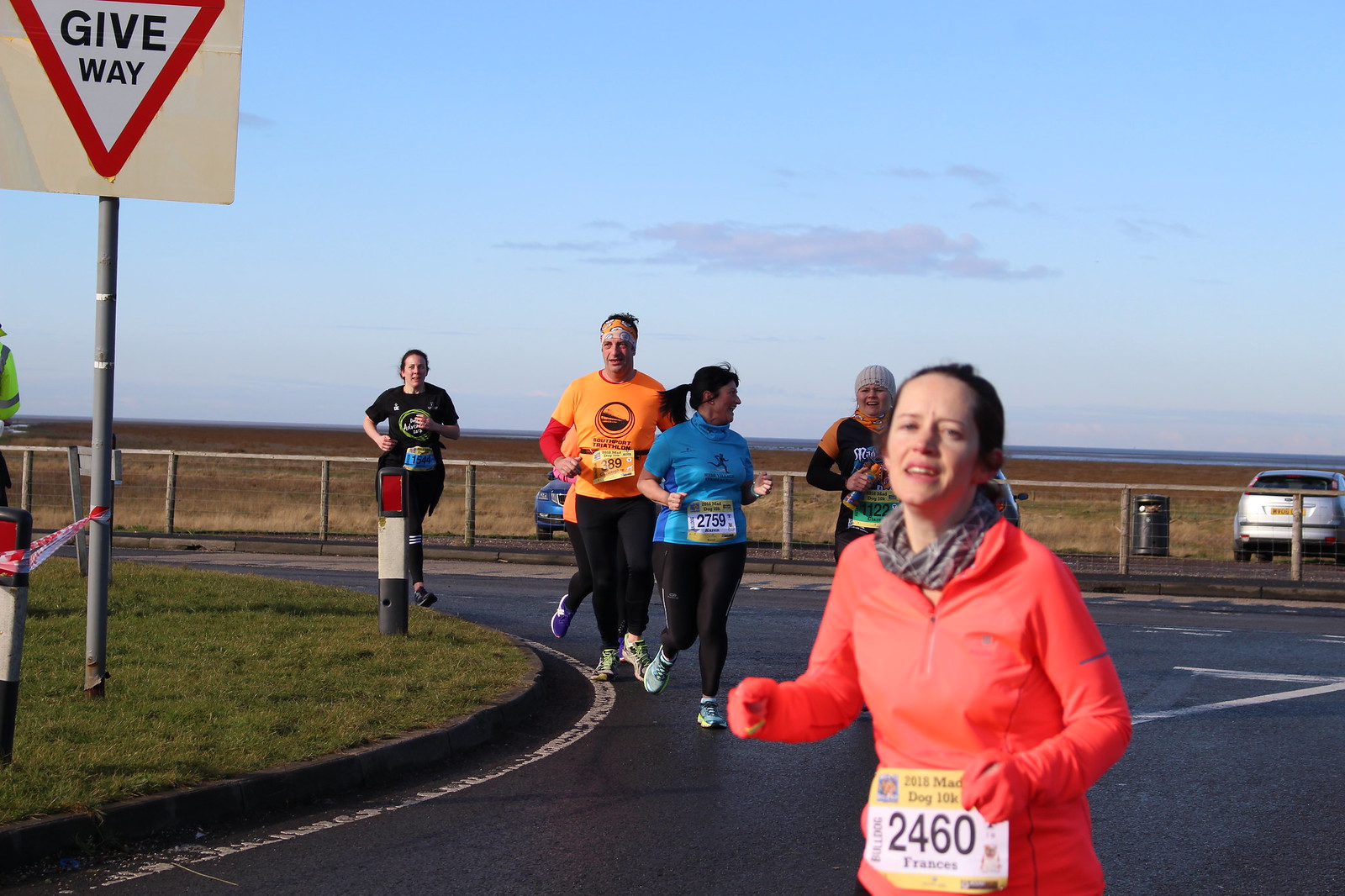In this vibrant and dynamic photograph captured during a daytime marathon, five runners are captured mid-stride as they navigate a bend in the road. The image is a horizontal rectangle with a well-balanced composition. 

In the top left corner, a "Give Way" traffic sign signals the impending curve. Just below this sign, a patch of lush green grass provides a natural contrast to the runners’ vibrantly colored attire. The sky, a brilliant blue, stretches across the top of the image, hinting at fair weather.

The most prominent runner occupies the bottom right corner of the photograph, her image captured from the waist up. She wears a light blue top and looks determined as she leads the pack. Behind her, the other four runners are partially visible, their athletic forms in various shades of orange, yellow, blue, black, and red. One runner sports a race bib with the number "2016" and the inscription "Bulldog 2460 France," indicating the event's competitive spirit and international participation. 

The overall scene exudes energy and movement, encapsulating the spirit of the race and the camaraderie of the participants, set against the backdrop of an outdoor marathon event.